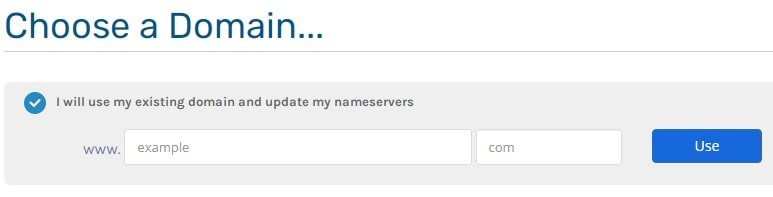This detailed caption vividly describes the image: 

The landscape-oriented image portrays a web page primarily set against a white background with no defined borders. At the top, bold bluish-green text prominently reads "Choose a domain...". Directly below, a thin grey horizontal line spans across the page, acting like a header. Beneath this line, there is a significant amount of white space followed by a long rectangular grey box with rounded edges. Inside this grey box, on the top left, a blue circle with a white checkmark is displayed, accompanied by black text that states, "I will use my existing domain and update my name servers."

Below this text, there is a grey “www” followed by two white boxes—the first one being longer and rectangular with "example" written inside it, and the second, smaller one displaying "com". To the right of these boxes, there is a blue rectangular button with rounded edges, longer than it is tall, featuring white text that reads "Use". This button seems intended for domain usage actions.